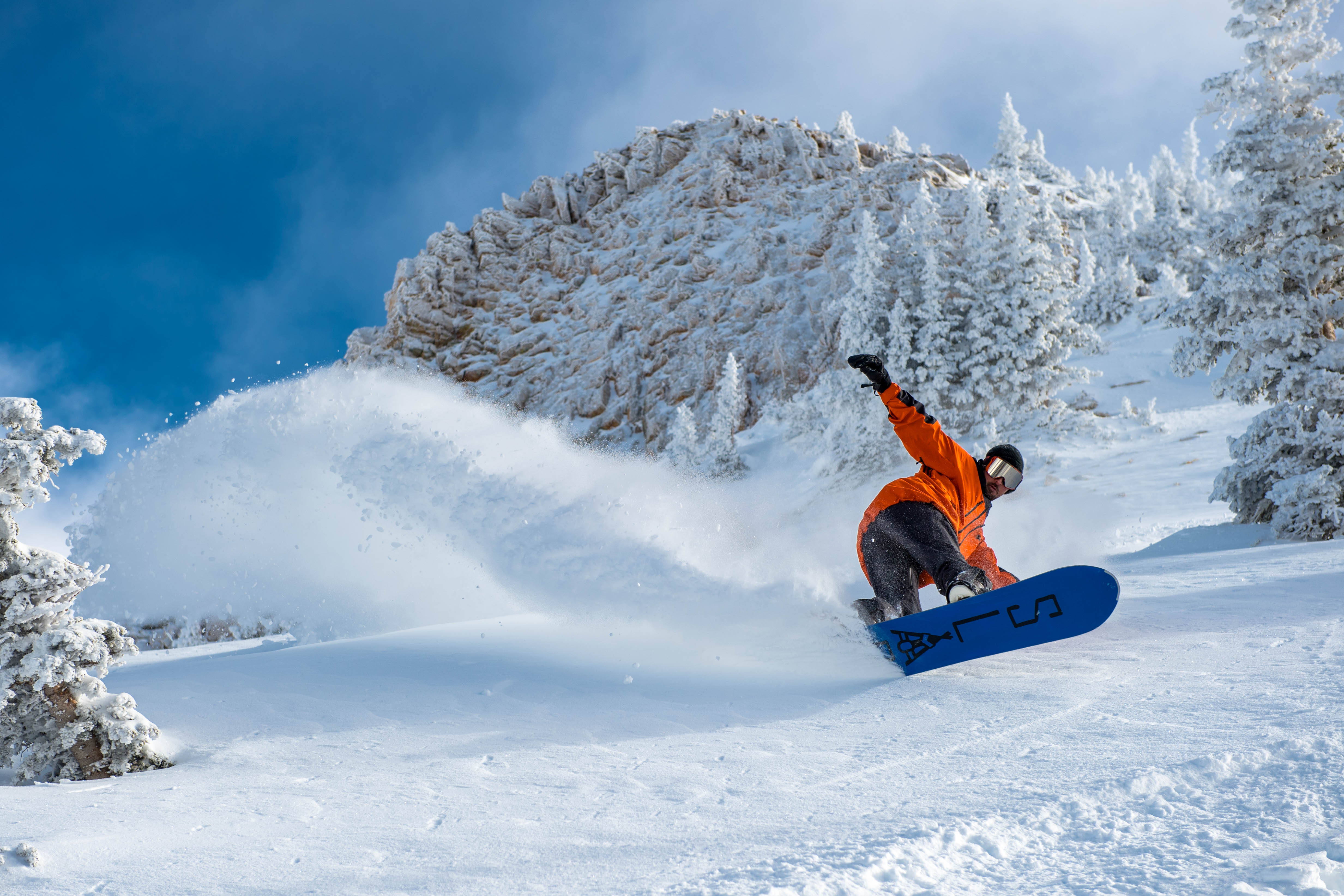A thrilling photograph captures a snowboarder carving down a picturesque mountain slope on a bright, sunny day with clear blue skies. The solitary figure is dressed in a striking orange winter jacket, black pants, black gloves, and a black hat, with silver-tinted goggles shielding his eyes. The snowboarder is mid-maneuver, with his knees bent and body curved, sending a flurry of snow into the air behind him. He rides a blue snowboard, the underside of which prominently features the word "SLIM." The scene is set against a breathtaking backdrop of snow-covered pine trees and distant snow-capped peaks, evoking a serene yet exhilarating winter landscape.